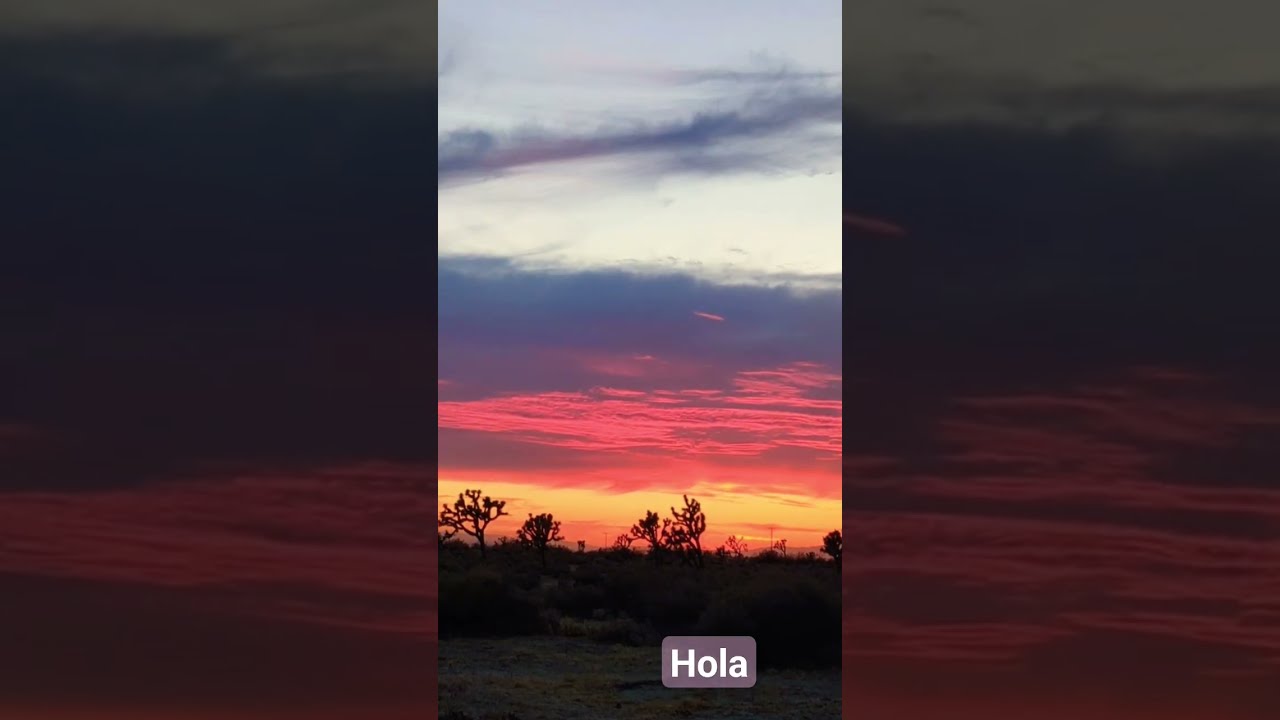The image, taken vertically like on a cell phone, is divided into three equal rectangles. The central rectangle features a dramatic sunset. The sky transitions from a light grayish-blue at the top, to dark gray, then a blend of ombre purples, reds, oranges, and finally a bright yellow and orange at the bottom. Silhouettes of trees and bushy terrain with dirt patches are visible in the foreground. Beneath the sunset photo, a highlighted block displays the word "Hola" in white font. The rectangles on either side of the central image are darkened, appearing black, framing the vivid sunset scene.